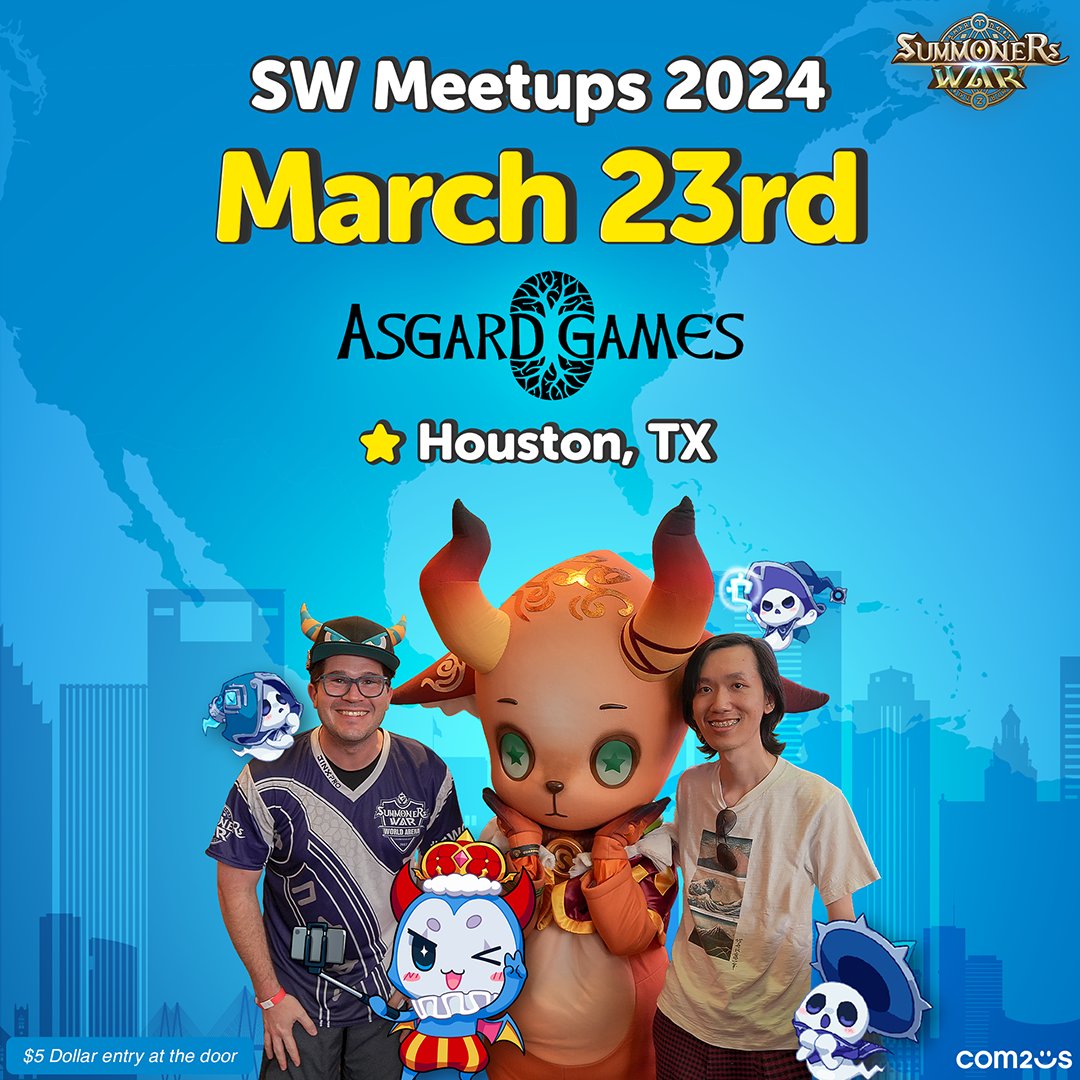The image is a color photograph in a square format, serving as an advertisement for the "SW Meetups 2024" event. At the top center, white text reads "SW Meetups 2024," followed by "March 23rd" in large yellow letters, and "Asgard Games" in black text with an elliptical logo featuring tree branches above and roots below the text. Below this, "Houston, Texas," is written in white letters accompanied by a yellow star pinpointing Houston's location on a blurred map in the background. The top right corner features the logo for "Summoner War."

Central to the photograph are two young men standing on either side of a character figure with a cat-like head, adorned with large curved horns and metal engravings. The character's eyes are light blue with dark blue stars. The man on the left is dressed in a dark blue/light blue jersey with a shield logo on the chest, a dark blue hat with angry blue eyes and multicolored horns, dark glasses, dark shorts, and is smiling at the viewer. The man on the right is an Asian young man in a white t-shirt featuring a vertical series of three graphics, wearing checkered pants or shorts, with long dark hair.

Surrounding the figures are various cartoon characters, including white ghosts with blue hats and different expressions. Among these is a blue cat-like cartoon character with a red crown and red and gold pantaloons, located at the bottom left, winking at the viewer. The background also features an animated blue city skyline with smoke pillars. 

The bottom of the image includes additional text: "5 dollar entry at the door" on the left in white, and "Com2Us" on the right in white text. The style of the image blends photographic realism with elements of graphic design.